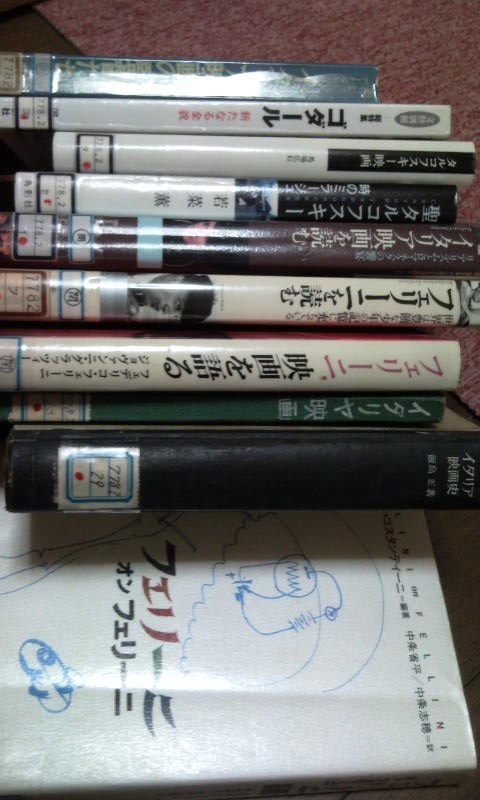This photograph showcases a stack of ten items, possibly DVDs, game CDs, or books, featuring Asian, likely Japanese, writing on their covers. The image appears to be taken in an amateur setting inside a home, illuminated by either a camera flash or natural light from a nearby window. Positioned on a dark reddish or maroon background, the items are stacked horizontally. 

Starting from the bottom, the lowest item features a white cover adorned with blue creatures and text. Directly above it is a thick black box, followed by items in green, cream white with black writing and pink accents, another white cover with a face illustration and black text, a colorful design in brown with blue and black elements, a black and white cover with blue accents, a white cover with black insertions, and a brightly lit green box at the very top. The angular perspective of the photograph suggests the need to rotate the image 90 degrees to view the stack in a straightforward manner.